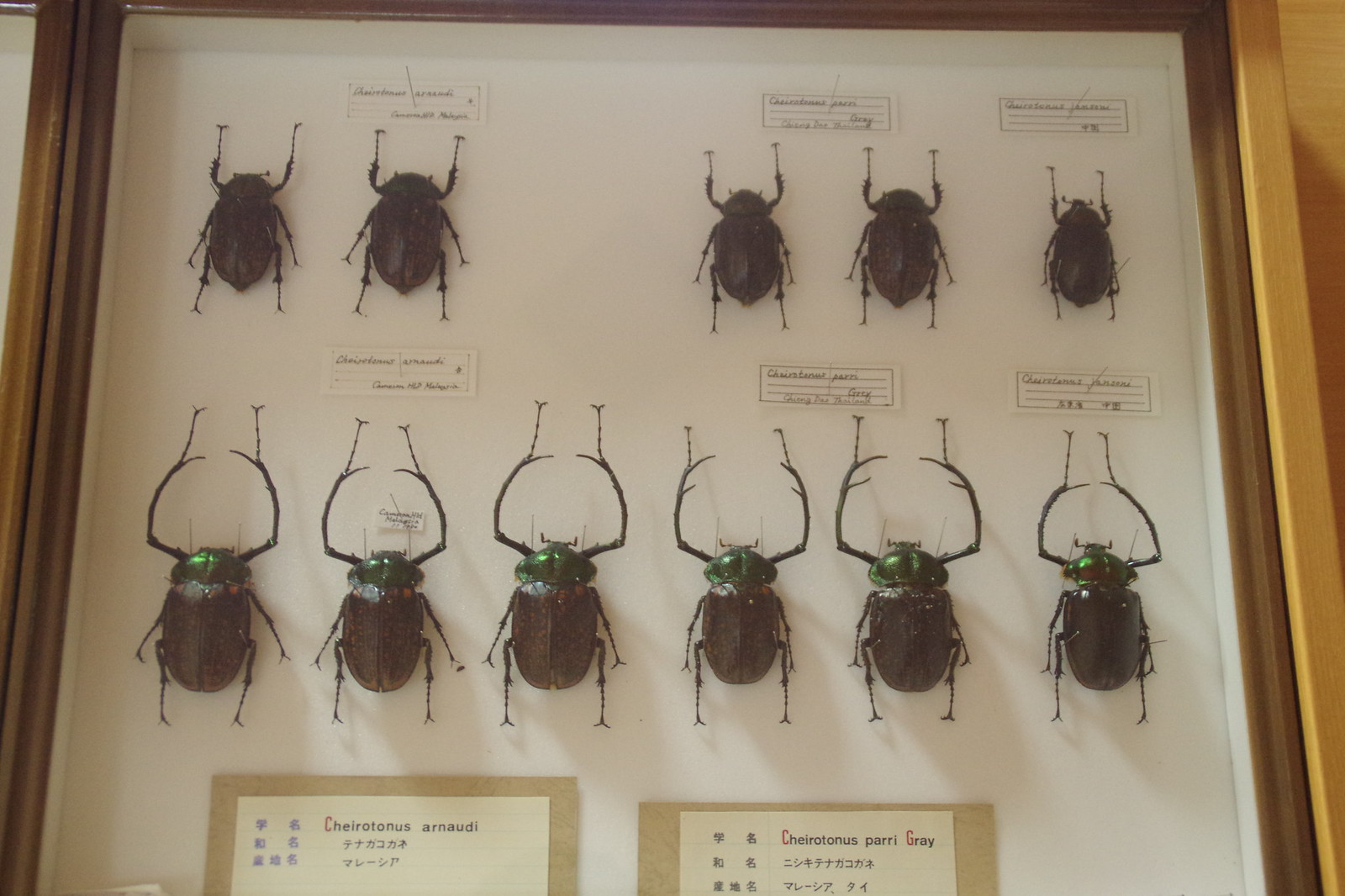The picture showcases a meticulously arranged entomology display within a double-framed mounting, surrounded by a white and light brown background. The central frame is dark brown, encapsulating a white board adorned with pinned beetles for preservation and identification. The board includes various labeled sections, providing details about the different beetles.

In the upper left corner, two beetles are positioned, while the upper right hosts three more. These insects are characterized by their uniform black bodies. The lower section displays six larger beetles with dark bodies and distinct green heads or thoraxes, notable for their long, curved antennae reminiscent of incomplete circles. These larger beetles feature prominent legs or clasping arms extending outward, highlighting the intricate details of their anatomy. The display is covered with glass, ensuring the preservation of the beetles and the clarity of the descriptive labels positioned above and below each specimen.